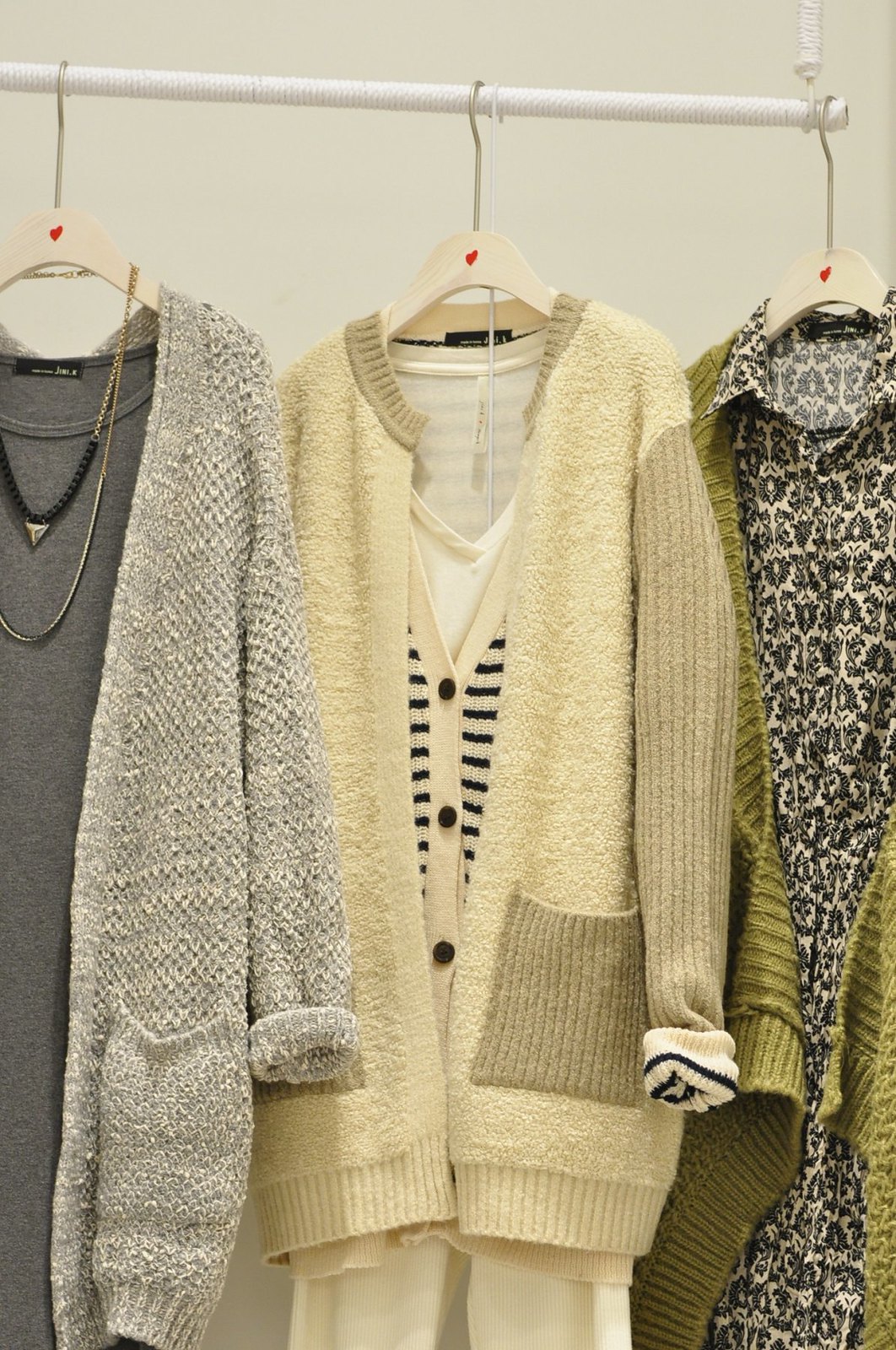This photograph showcases a neatly organized closet with a white background, where three distinct outfits are hanging on wooden hangers, each adorned with a red heart. These hangers are suspended from a horizontal white clothes pole wrapped in twine or thin white rope. 

On the left, there's a dark, scoop-neck cotton dress, complemented by two looped necklaces. Over it, a loose-knit gray cardigan without buttons drapes down to about mid-thigh. In the middle, a cream-colored outer cardigan with brown pockets, sleeves, and collar covers a long white t-shirt, giving the appearance of pants hanging below. This ensemble includes a V-neck t-shirt layered under a striped cardigan. The rightmost outfit features an olive green cardigan extending beyond the waist, layered over a collared shirt with an abstract black-and-white design on a cream background. The shirt appears to have a length suggesting it could be a dress. Each piece is meticulously arranged to highlight the textures and colors, providing a harmonious display within this retail setting.